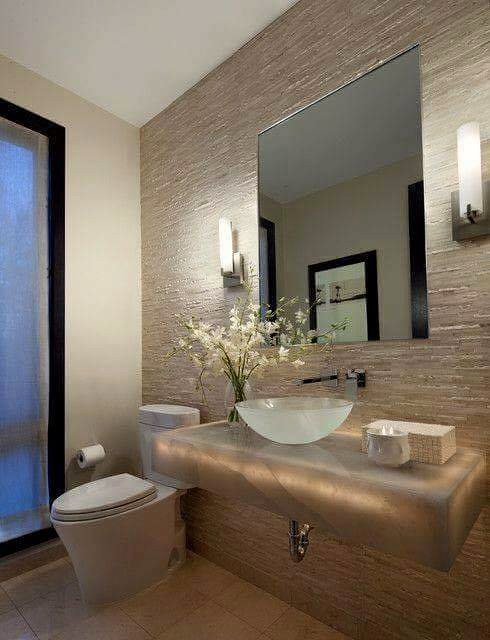In this luxurious bathroom, the focal wall boasts beautifully textured tiles that resemble rock with a golden hue. A frameless mirror is mounted above a sleek, metallic countertop, perfectly centered between two elegant wall sconces on either side. Beneath the mirror, a sophisticated glass bowl sink extends from the counter, which adds a modern touch to the space. Beside the sink, a delicate jar of jasmine flowers adds a touch of nature and freshness.

To the right of the sink, a white candle and a box of tissues are neatly arranged for convenience. Adjacent to this setup, a pristine white toilet is positioned against a green-painted wall. The bathroom features an almost floor-to-ceiling, black-framed window with an opaque pane, allowing soft natural light to diffuse through the room while maintaining privacy. This harmonious blend of textures, colors, and essential elements creates a serene and elegant atmosphere in the bathroom.